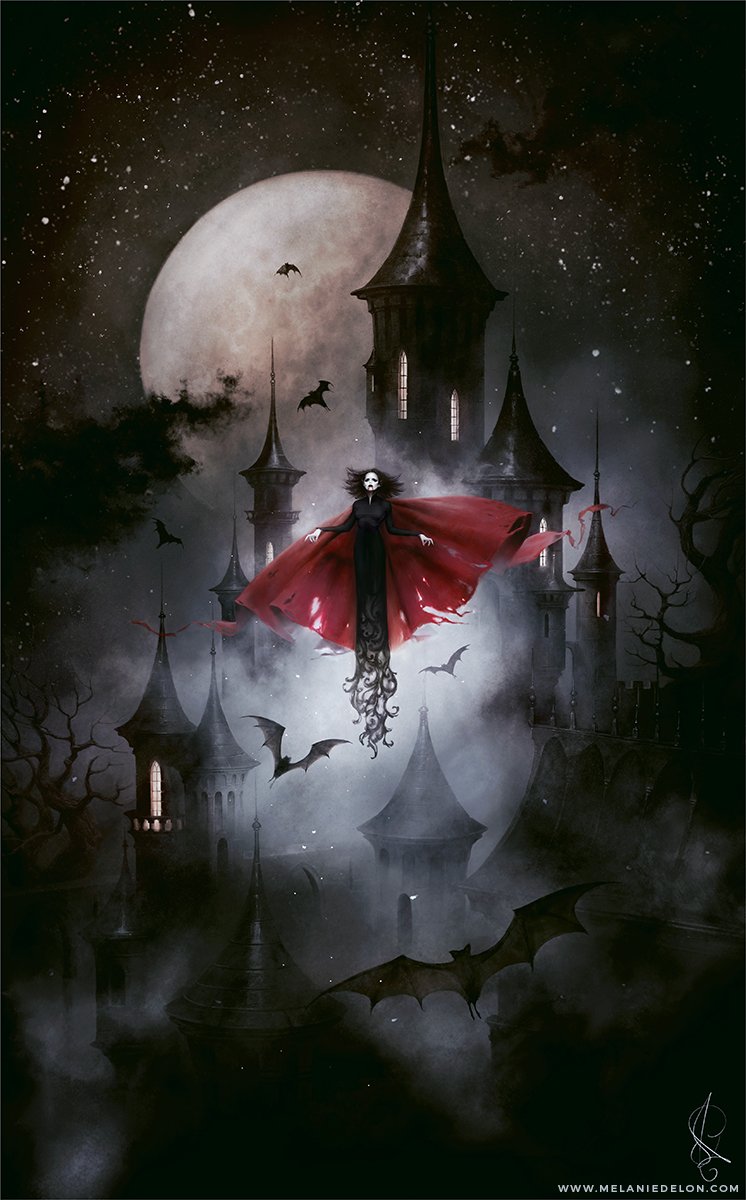In this evocative nighttime scene, the image strikingly resembles a painting, featuring an ominous, black star-dotted sky dominated by a large, partially obscured full moon. The moon's ethereal glow highlights a towering, multi-tiered castle whose dark silhouette pierces the night with several steeples, partially shrouded in fog and smoke that seem to breathe life into the mystic atmosphere. At the forefront, a spectral figure, reminiscent of a vampire, commands attention. Clad in a flowing dark red cape and an equally dark outfit, the figure's white face and wind-swept hair add to the eerie, Halloween-like ambiance. Surrounding this figure, numerous black bats punctuate the air, creating a sense of movement and adding to the haunting tableau. Amidst this atmospheric scene, the website www.melaniedlon.com is subtly inscribed in the bottom right corner, grounding the otherwise surreal visual.